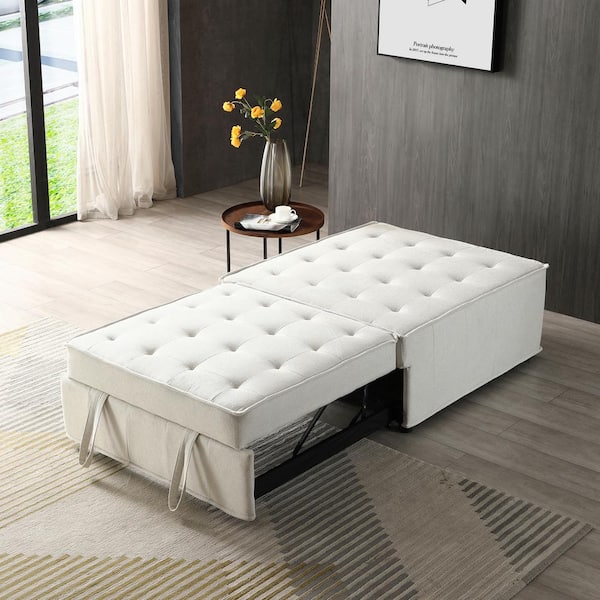This detailed photograph captures a stylish and multifunctional living room. The room features light brown wooden flooring and grayish wood-paneled walls, complemented by light gray baseboards. In the center, there is a rug with an interesting pattern of brown and light green stripes, interspersed with gray. Dominating the room is a versatile, upholstered settee that can be pulled apart to double in size, transforming into a flat seating area or even a single bed. This furniture piece, covered in a white or faux leather material, has visible handles which facilitate its transformation back into a compact ottoman. Nearby, a small circular table holds a cup of espresso and a vase with vibrant yellow flowers, likely black-eyed Susans. The room is brightly lit, thanks to a large floor-to-ceiling window or sliding patio door adorned with long, sheer beige curtains. This window offers a serene view of grass and a sidewalk, blurring the line between indoor and outdoor spaces.